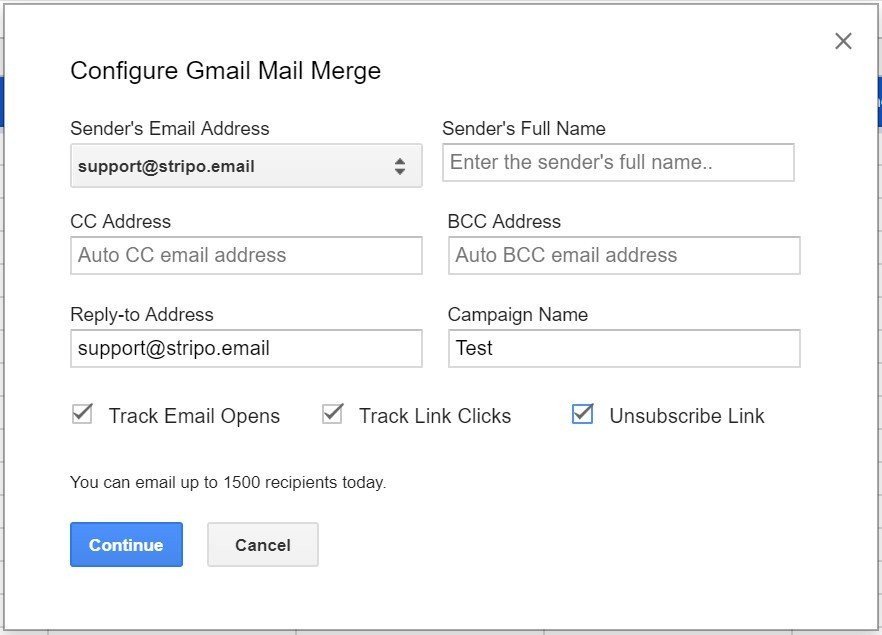A white rectangular interface, wider than it is tall, features a minimalist design with finely lined black borders. Positioned in the top left corner, the text "Configure Gmail Mail Merge" is clearly displayed. 

Directly below, the label "Sender's Email Address" is followed by an input field containing the email address "support@stripo.email." This field has a gray background and contains an up and down arrow to its far right, likely for additional settings or choices.

The next section reads "CC Address," with a placeholder text in the data field stating "Auto CC Email Address" in gray. Below this, the label "Reply To Address" is followed by another input field with the pre-filled email "support@stripo.email."

On the right-hand side, there is a label "Sender's Full Name," adjacent to which is a data field prompting the user to "Enter the sender's full name" in gray placeholder text.

Further down, an input section labeled "BCC Address" contains a field with "Auto BCC Email Address" grayed out as a placeholder. Following this, the "Campaign Name" field displays the text "test."

In a horizontal layout below these fields, there are settings for tracking email activities with labels: "Track Email Opens," "Track Link Clicks," and "Unsubscribe Links." Each of these options is accompanied by a checkbox, all of which are ticked.

At the bottom, a note informs the user, "You can email up to 15,000 recipients today." This message is followed by two buttons: a blue "Continue" button with white text and a gray "Cancel" button with black text. The interface includes an 'X' icon located in the upper right corner for closing the configuration window.

The color palette used in this interface includes shades of black, gray, blue, and white.